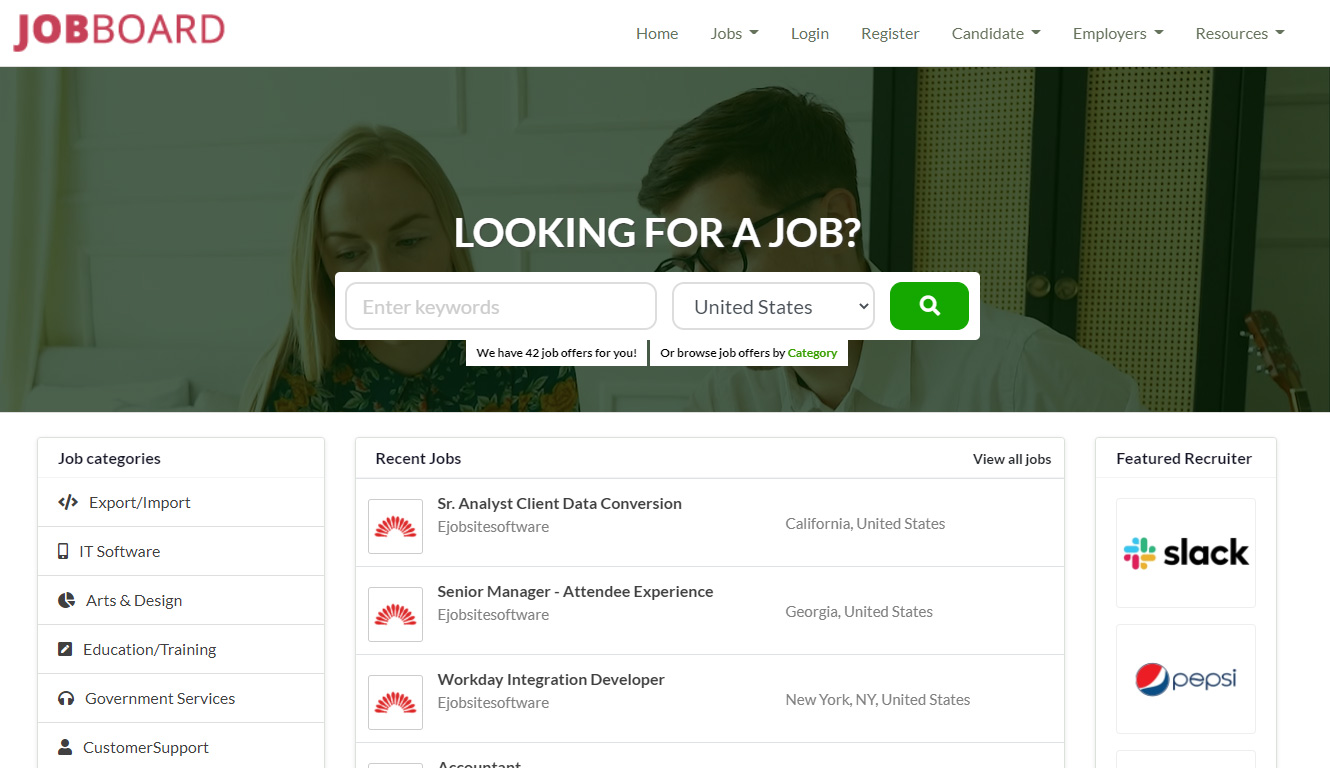In this image, the top and bottom portions are white. At the top, in bold red capital letters, it reads "JOB" followed by "BOARD" in a slightly less bold red font, showing the words in all caps without any spaces between them. 

Below this section, aligned to the far right, there are several navigation options: "HOME," "JOBS" (with a drop-down menu), "LOGIN," "REGISTER," "CANDIDATE" (with a drop-down menu), "EMPLOYERS" (with a drop-down menu), and "RESOURCES" (with a drop-down menu).

In the center of the page, taking up approximately one-third of the screen, there is a darkened rectangular image. Despite the dimness, the faces of a woman with straight blonde hair and a man are visible, seemingly searching for something. Overlaid on this image is a title in all caps, reading "LOOKING FOR A JOB?" in white text. Below this, there’s a section to "ENTER KEYWORDS" in a white text box, alongside a drop-down menu labeled "UNITED STATES." To the right, there is a green search button featuring a white magnifying glass icon, signaling to click when ready to search.